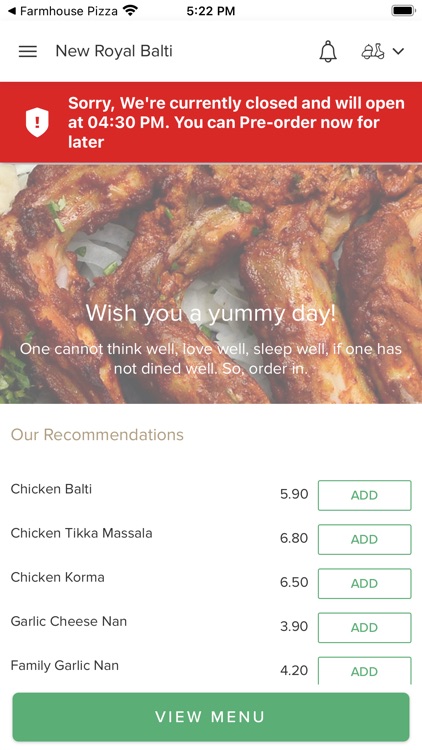Here's a cleaned-up and detailed caption for the image described:

---

**Screenshot Description: Farmhouse Pizza Mobile App** 

The image is a screenshot of the Farmhouse Pizza mobile app, displayed on a white background. 

- **Header Section:**
  - **Top Left:** The app name "Farmhouse Pizza" is prominently displayed in bold black letters. An arrow pointing to the left, located to the left of the text, provides a way to return to the homepage.
  - **Top Right:** A menu icon, displayed in black, is positioned to the left of the text "New Royal Balti," also in bold black letters. Adjacent to this are an alert icon and an additional dropdown icon for further options.

- **Status Banner:**
  - Below the header, a red banner states, "Sorry, we're currently closed and will reopen at 4.30 p.m. You can pre-order now for later."

- **Promotional Section:**
  - A vivid image of chicken wings is presented, with an inviting text overlay: "Wish you a yummy day. One cannot think well, love well, sleep well if one has not dined well, so order in."

- **Recommendations Section:**
  - A gray subtitle reads "Our Recommendations," followed by a list of recommended dishes:
    - **Chicken Balti**
    - **Chicken Tikka Masala**
    - **Chicken Korma**
    - **Garlic Cheese Naan**
    - **Family Garlic Naan**
  - Each dish's name is accompanied by its price and an "Add" button, located at the far right of each item.

- **Footer Section:**
  - A green button at the bottom of the screen invites users to "View Menu."

---

This caption provides a detailed and organized description of the user interface elements in the Farmhouse Pizza mobile app screenshot.